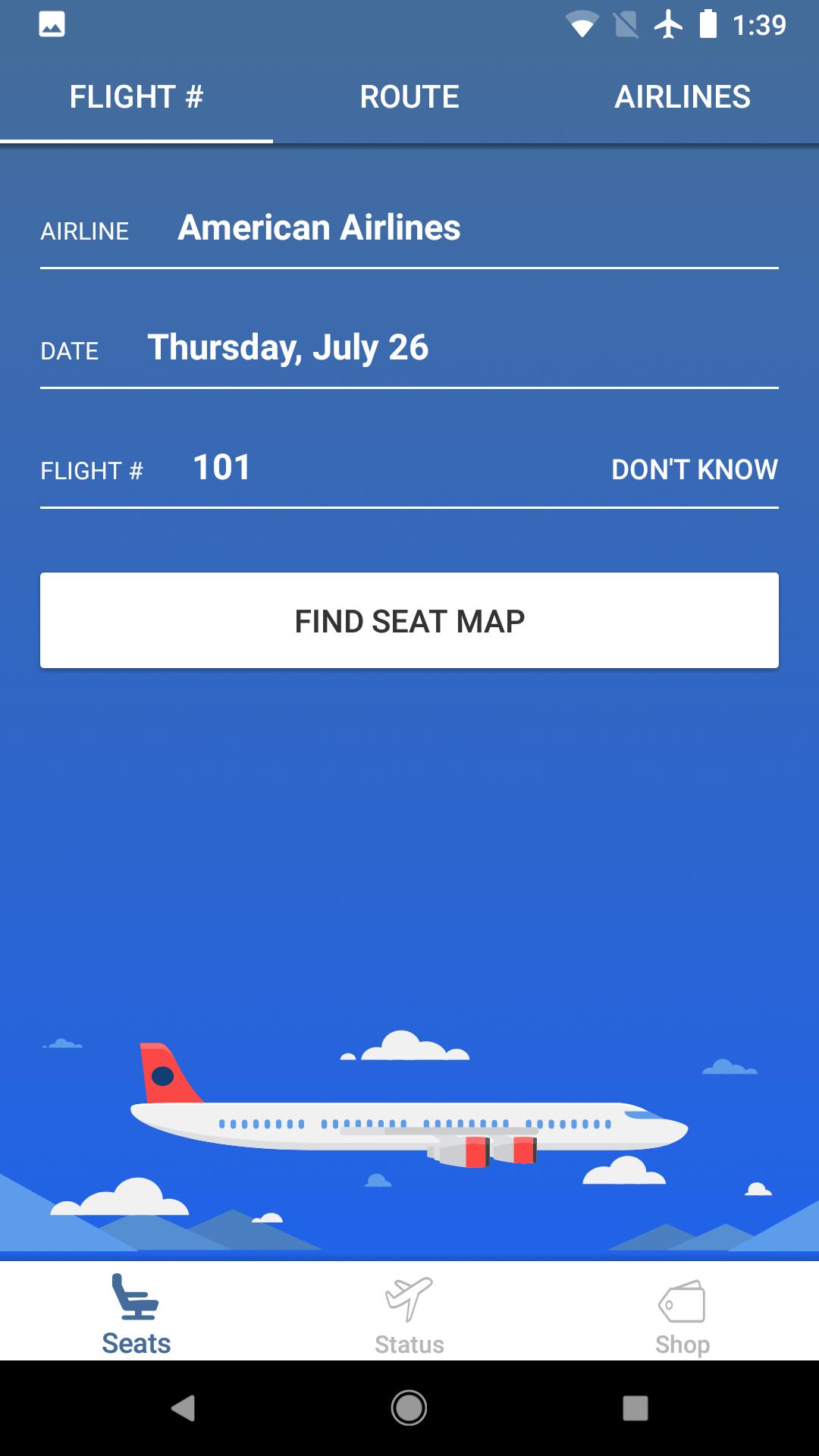Caption: 

An in-flight informational screen for American Airlines Flight 101, traveling on Thursday, July 26th. The top portion of the screen features a playful cartoon image of a white airplane soaring through a blue sky dotted with fluffy white clouds. Below the image, the user interface includes several sections: 

- **Status Bar:** Depicts the flight number, route, and airline details, all written in white against a blue background.
- **Navigation Options:** Features icons for "Seats," "Status," "Shop," and navigation buttons including a back arrow, a circle, and a square.
- **Borders:** The bottom of the screen is edged with a black border, topped by a narrower white border.

The overall design is predominantly blue with white text, ensuring clear visibility and easy navigation for passengers. The information is supplemented with additional elements like a map for finding seats and a status update on various flight amenities such as Wi-Fi and in-flight entertainment. 

(NASA Jet Propulsion Laboratory and the California Institute of Technology are mentioned, but their relevance to the image is unclear and may not be directly related to the flight screen.)